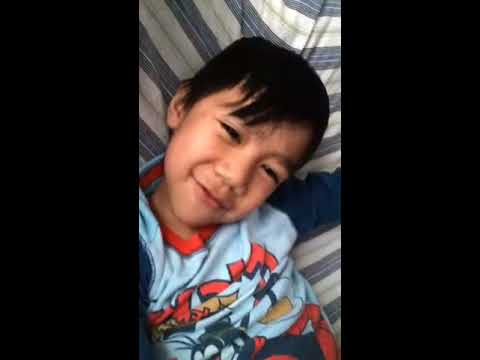In this image, we see a young, likely three or four-year-old Asian boy with black, slightly messy hair that is parted to the side with bangs. He is sitting comfortably on what appears to be a bed or couch with white and gray striped upholstery or possibly a matching blanket. The boy is dressed in a light blue shirt adorned with dark blue sleeves and an orange-red collar. The shirt features a cartoon graphic that could be reminiscent of a character like Daffy Duck, along with some orangish script. The boy's expression is one of joy; his head is tilted, he is smiling broadly, and he appears to be singing or telling a joke. The overall scene suggests a sunny, cheerful day, as the boy is clearly enjoying the moment.